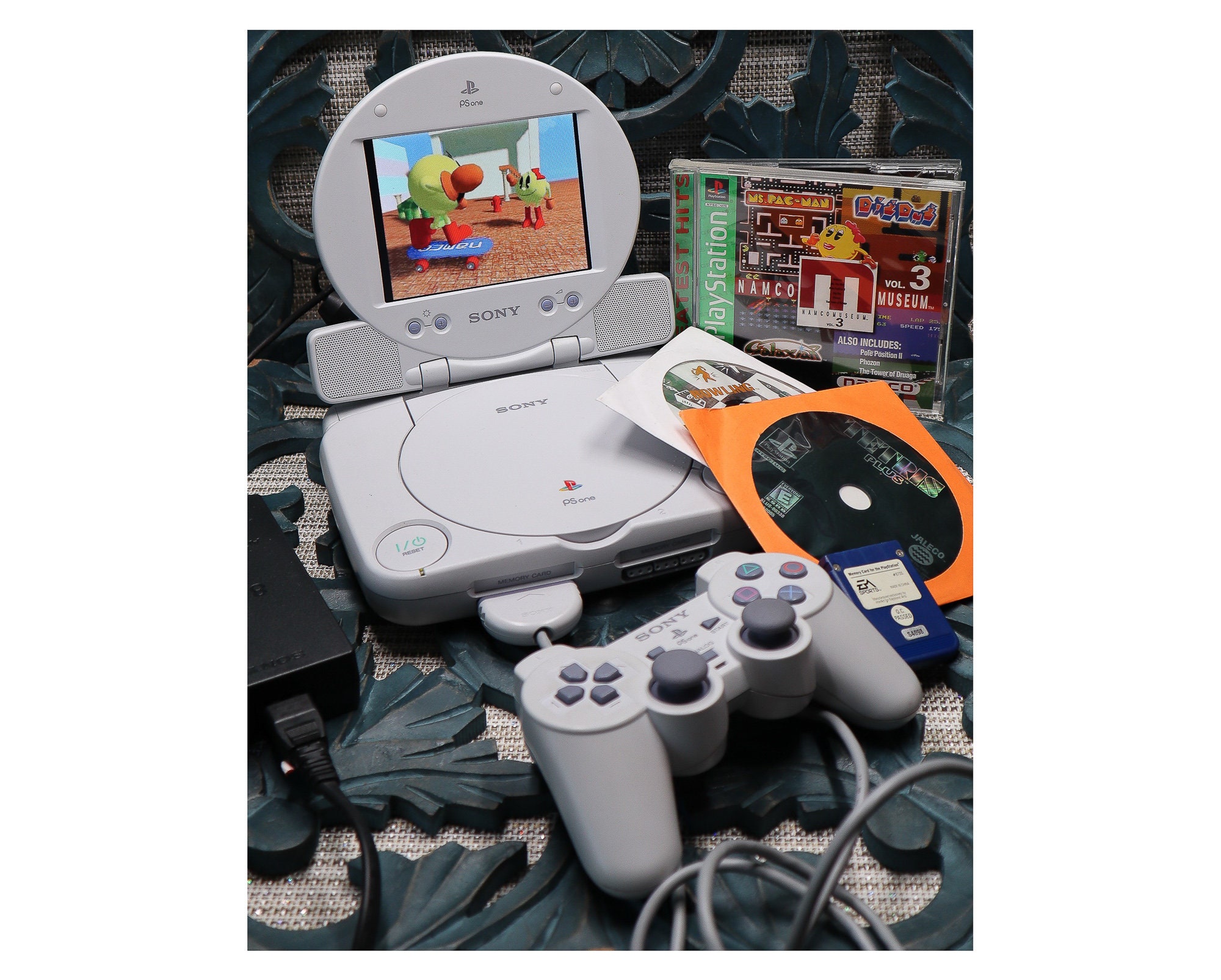This photograph features a vintage Sony PlayStation 1 gaming console, distinguished by its gray color and compact design. The focal point of the image is the console itself, which has a unique circular screen attachment complete with integrated speakers, set above the console's disc tray. A classic gray PlayStation controller is connected to the console, lying in front of it. 

Several game discs are scattered beside the console: in the top left corner, a distinctive Ms. Pac-Man CD is visible, while to the right, there are two other game discs—one in an orange case and another in a white case. One of these discs appears to be Tetris, while the title of the other remains unreadable.

Centrally placed on top of the CDs to the right is a purple memory card featuring the EA Sports logo. Additionally, there’s a black charging cable visible on the left side of the image. The overall setup evokes a strong sense of nostalgia, highlighting the iconic era of the original PlayStation gaming experience.